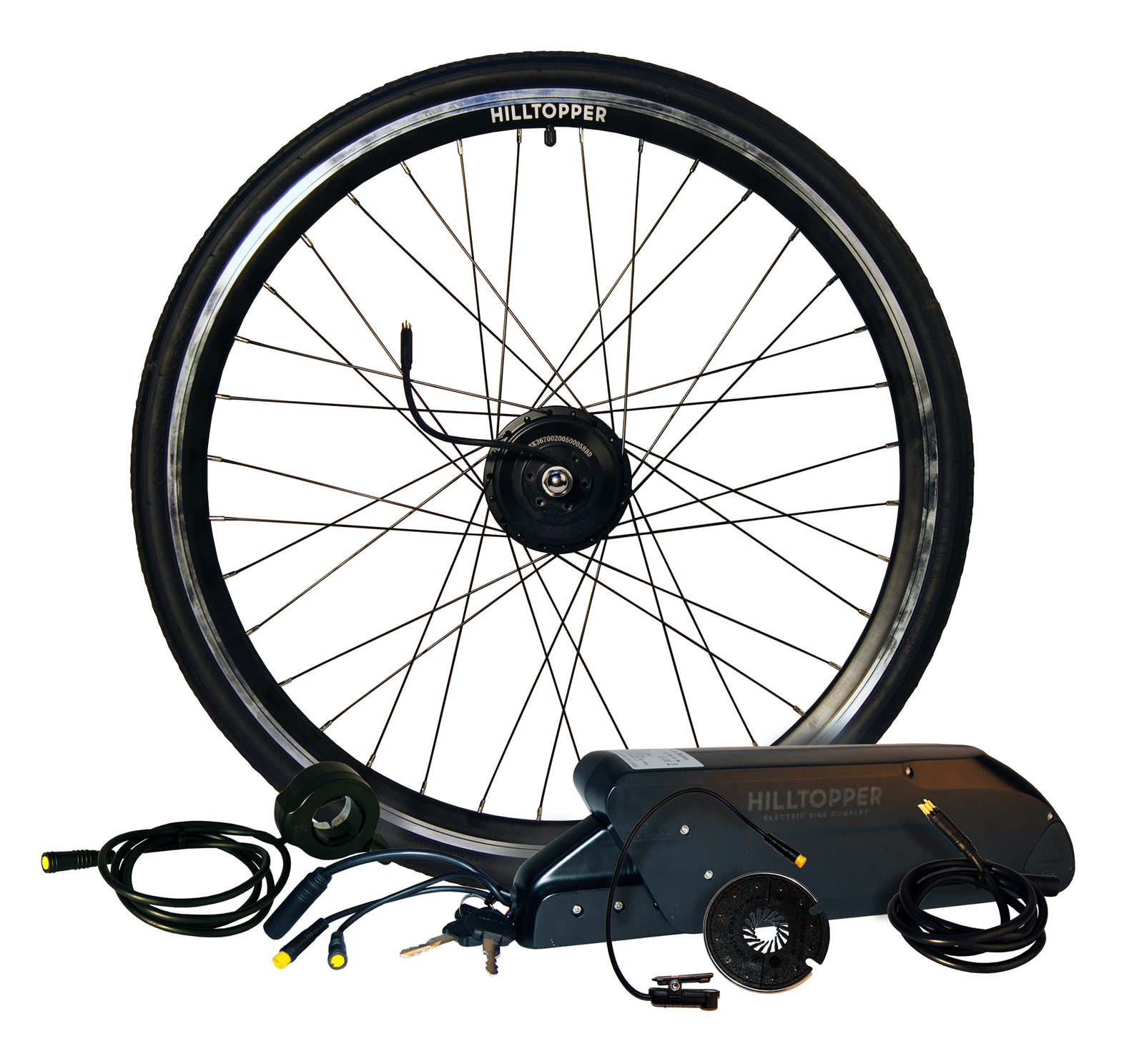The image showcases a close-up of a black rubber bicycle wheel, prominently branded with "Hill Topper" in white print on its shiny silver rim. The wheel features a cross-spoked design and has an electrical cord emanating from its center. Accompanying this setup, various accessories are visible on the ground beneath the wheel, including a set of keys, some connectors, and an oblong black box labeled "Hill Topper Electric Bike Company" with a white label. The tire appears to be new, with a pristine rubber surface and gleaming silver metal parts, suggesting it might belong to an electric bike system.